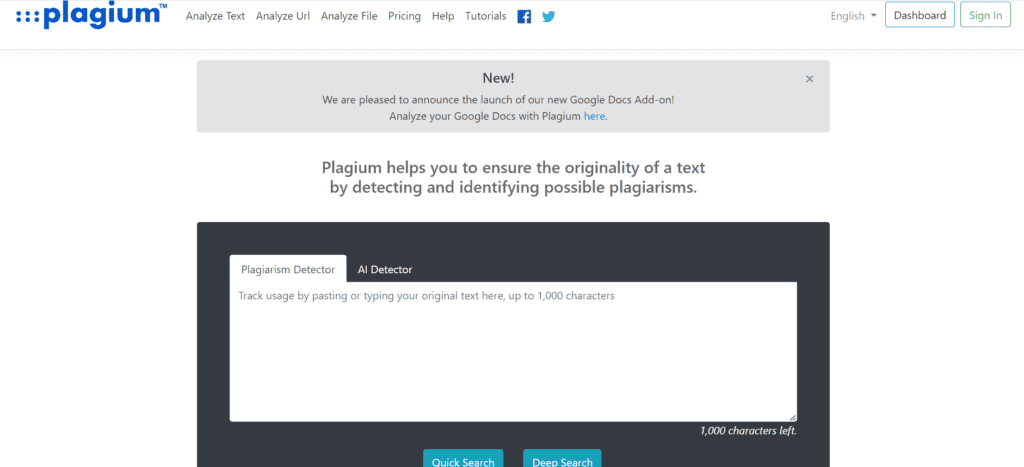The image displays a screenshot of a webpage from Plagium, a plagiarism detection service. In the upper left corner, the Plagium logo is prominently featured, which consists of the company name in blue text and six polka dots to its left. Below the logo, there is a centered gray box with the text: "We are pleased to announce the launch of our new Google Docs add-on. Analyze your Google Docs with Plagium here," with the phrase "here" being a clickable blue link.

Underneath, there is a black rectangular box with a white inner section. This section contains text instructing users to "Track usage by pasting or typing your original text here up to 1,000 characters." Below this instruction, there are two blue action buttons labeled "Quick Search" and "Deep Search," allowing users to choose between different levels of plagiarism detection.

Overall, the image effectively showcases the primary features and instructions for using Plagium's new Google Docs add-on.